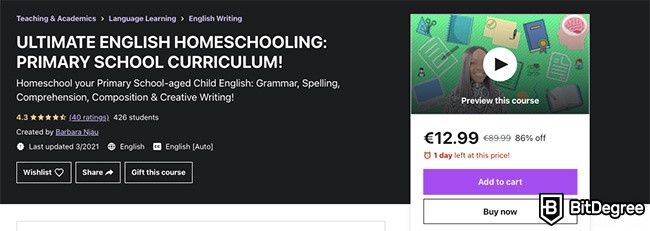This is a detailed caption for an educational course screenshot:

At the top of the screenshot, a large black rectangle spans the width of the image. In the upper left-hand corner, gray text reads "Teaching and Academics." Following this label, a right arrow (sideways "V") points towards the next category: "Language Learning," followed by another right arrow leading to "English Writing."

Several lines below, large white text in all caps announces: "ULTIMATE ENGLISH HOMESCHOOLING: PRIMARY SCHOOL CURRICULUM!" In smaller white text below, the subtitle reads, "Homeschool Your Primary School-Aged Child in English: Grammar, Spelling, Comprehension, Composition & Creative Writing."

Beneath this text, a rating system with stars is followed by the creator's name and the last updated date. Further down, three outlined buttons in white are displayed: the leftmost button is labeled "Waitlist" with a heart icon, the middle button reads "Share" with an arrow, and the rightmost button says "Gift this Course."

On the right side of the screenshot, a green rectangle at the top displays a variety of colored books and a picture of a woman. In the center of this section, a white circle with a play button (right-pointing arrow) prompts users with "Preview the Course." Below this preview prompt, the price of the course is listed in white, followed by two buttons: a purple "Add to Cart" button with white text and a white "Buy Now" button outlined in gray with black text.